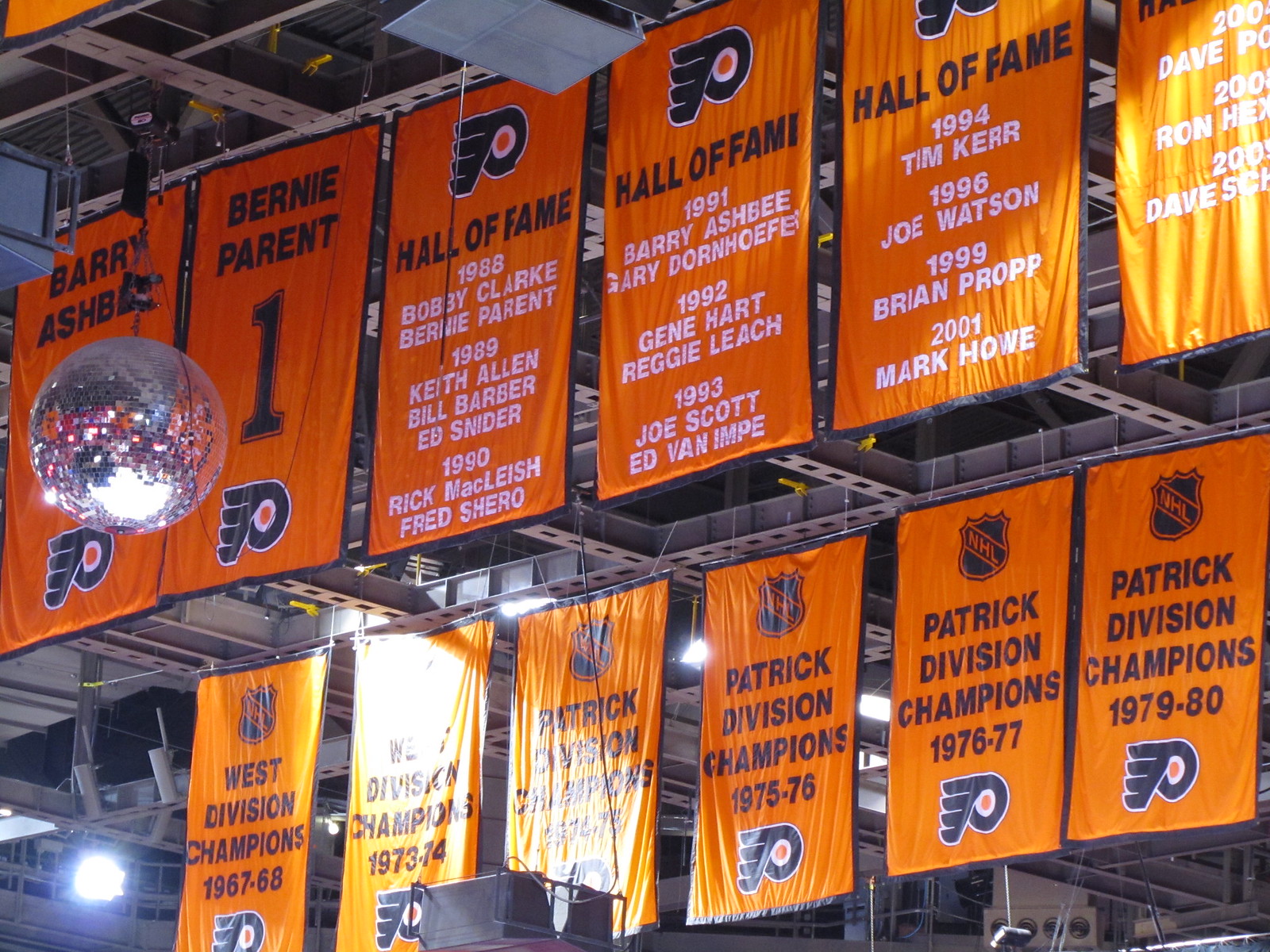The photograph captures the interior of the Philadelphia Flyers hockey rink, focusing on the ceiling rafters and the array of banners suspended from them. The prominent metallic gray rafters support a series of vibrant orange banners, each featuring the iconic Philadelphia Flyers logo—a stylized 'P' resembling a hockey puck with wings to the left. In the upper left-hand corner of the image, a large disco ball adds an unexpected reflective shimmer to the scene.

The banners are arranged in two rows. The first row includes individual player honors, starting with Barry Ashby and Bernie Parent, who is denoted with his number one. This segment also displays banners honoring Hall of Fame inductees: Bobby Clarke, Bernie Parent, Keith Allen, Bill Barber, and Ed Snider. Further to the right in this row are additional honored players: Rick MacLeish, Fred Shero, Gary Dornhoefer, Gene Hart, Reggie Leach, Joe Scott, David Van Impe, Tim Kerr, Joe Watson, Brian Propp, and Mark Howe, each with their respective induction years, although some names and years seem less legible and may overlap.

The second row beneath features six more banners marking significant team achievements. The banners on the far left commemorate the Flyers' Division Championships from the 1967-68 and 1973-74 seasons. The center banner is obscured by bright light, making it unreadable. The three banners to the right highlight the Flyers' Patrick Division Championships from the 1975-76, 1976-77, and 1979-1980 seasons.

This detailed and organized view of the rink's decor vividly showcases the storied history and celebrated achievements of the Philadelphia Flyers.